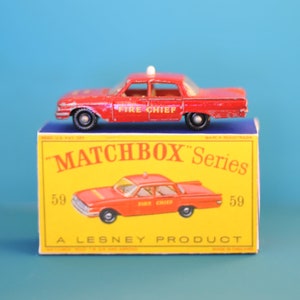The image features a vintage Matchbox toy car packaging set against a sky-blue background. The package, presented as a rectangular prism, showcases distinct design elements. The top part of the packaging is blue, while the viewable front part combines yellow as the dominant color, complemented by vibrant red text and artwork. 

The text at the top prominently reads "Matchbox Series" in red. Just below, the number "59" is displayed alongside an illustration of a red, 1950s-era car, specifically indicative of a model akin to what is colloquially referred to as a "hooptie." Beneath the car illustration, the phrase "A Lesney Product" is inscribed in black.

The car itself, depicted in red with "Fire Chief" written in white on its side, sports black tires with silver hubs. Additionally, a white light is positioned atop the car, signifying its emergency vehicle status. This detailed presentation effectively encapsulates the nostalgic essence of the collectible toy.